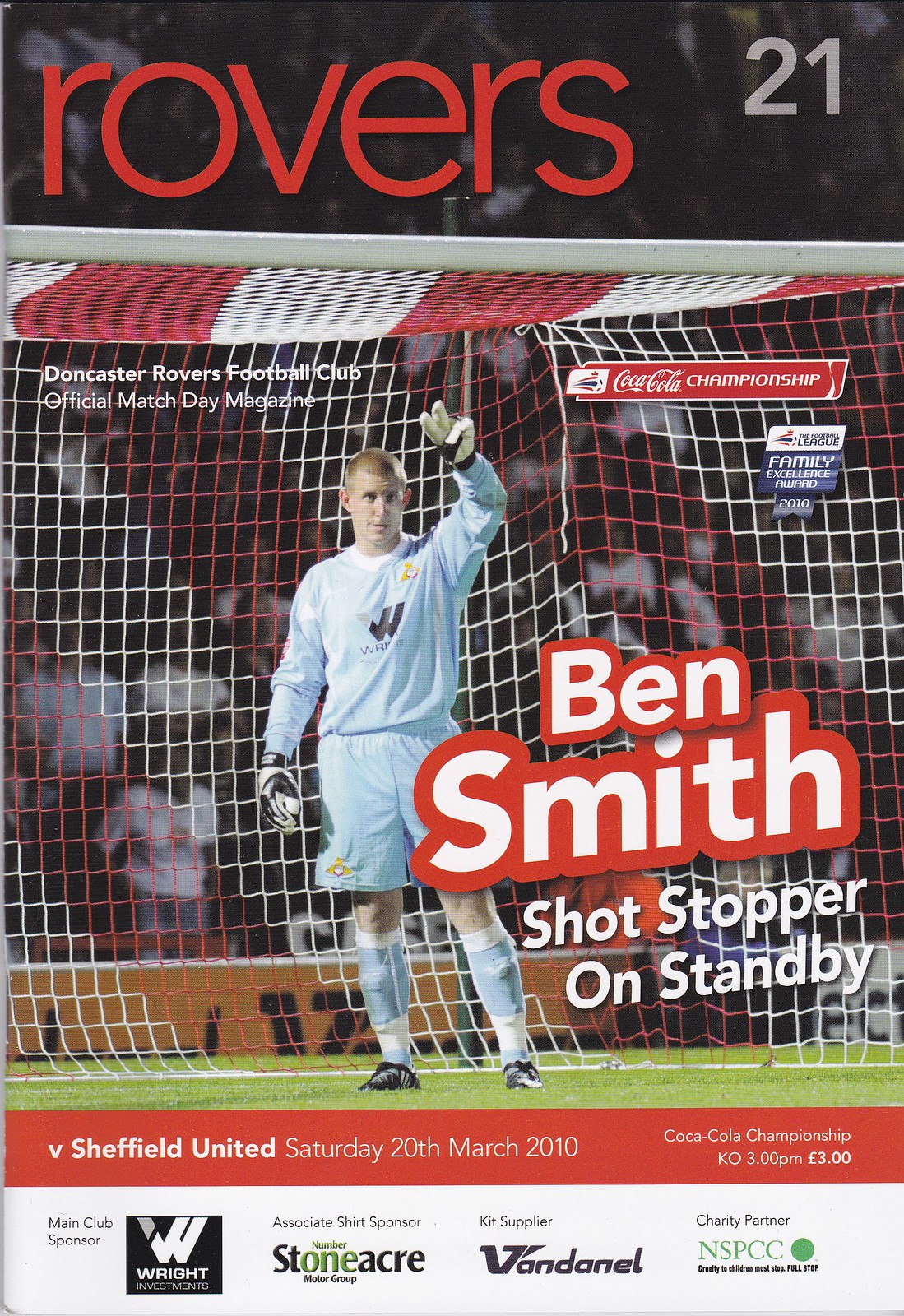This image portrays the front page of a sports magazine, showcasing a tall rectangular photograph of a soccer goalie, Ben Smith. The goalie is positioned centrally, sitting inside the goal, making a peace sign with his hand. He is dressed in a long-sleeve light blue and white uniform, with matching blue shorts and knee socks, alongside gloves, indicating his role. He has pale skin and short blonde hair. The net behind him features a striking pattern of thick alternating red and white stripes at the top and diagonal red and white stripes at the back, creating a dynamic background.

The top portion of the image includes a blurred, dark area, above which the magazine title "Rovers 21" is prominently written in red letters. Surrounding Ben Smith's image, white font encased in red borders reads "Ben Smith," followed by the phrase "Shotstopper on standby" in bold white letters. Further down, the page details "Doncaster Rovers Football Club, official match day magazine," though the full text is somewhat obscured. An eye-catching Coca-Cola advertisement appears to the right of the goalie. Additionally, a horizontal red bar spans the bottom, inscribed with "vs Sheffield United, Saturday, March 20th, 2010" and features multiple advertising logos.